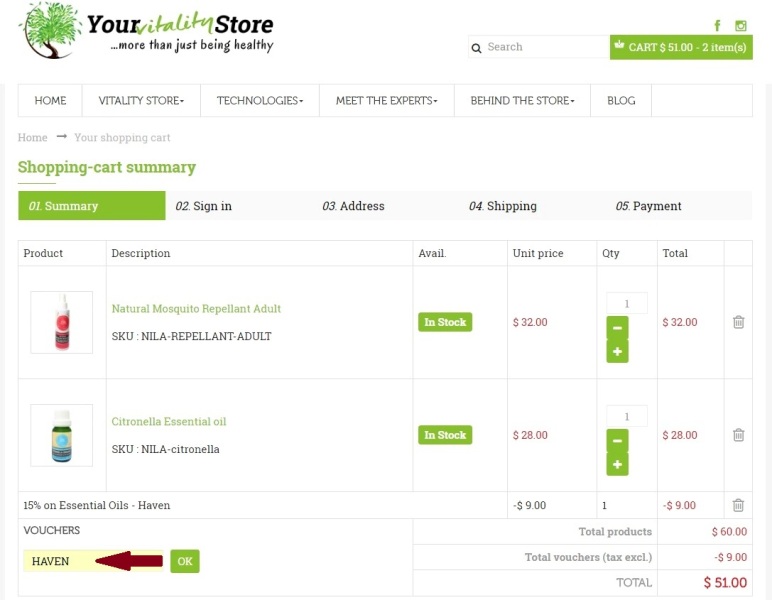Here's a refined and detailed caption for the screenshot:

"This screenshot showcases the homepage of 'Your Vitality Store'. At the top left, a circular logo features a tree with green leaves and a round trunk, accompanied by the site's name, 'Your Vitality Store', and the tagline, 'Calypso... more than just being healthy.' 

On the top right, there is a search box followed by a bright green 'Cart' button displaying '$51' for two items. Positioned above this button are icons linking to Facebook and Instagram. 

The header row includes links to 'Home', 'Vitality Store', 'Technologies', 'Meet the Experts', 'Behind the Store', and 'Blog', with dropdown menus available in all but 'Home' and 'Blog'. Below, breadcrumb navigation indicates the user is on the 'Home' > 'Your Shopping Cart' page.

The main page title, 'Shopping Cart Summary', indicates the shopping cart's progress stages, with 'Summary' highlighted in green. The stages include 'Sign In', 'Address', 'Shipping', and 'Payment'.

The cart currently holds two items: 
1. Natural Mosquito Repellent (Adult) priced at $32 per unit, and 
2. Citronella Essential Oil priced at $28 per unit.

A 15% discount on essential oils from 'Haven' provides a $9 reduction, adjusting the total from $60 to $51. Notably, a red arrow points to the activated 'Haven' voucher code at the bottom left."